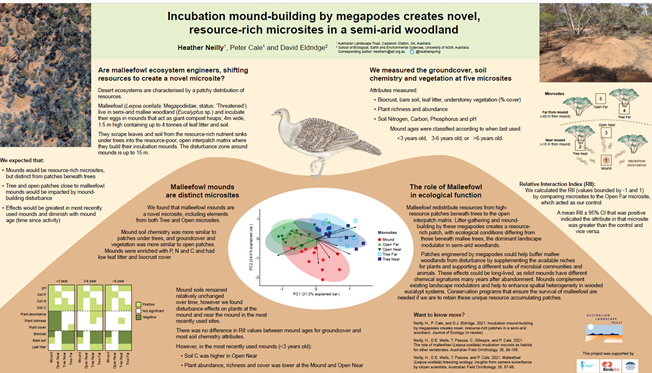The poster titled "Incubation Mound Building by Megapods Creates Novel Resource-Rich Microsites in a Semi-Arid Woodland" by Heather Neely, Porter Cole, and David Eldridge, presents a detailed scientific study. The research explores how megapod incubation mounds serve as unique microsites that enrich the ecosystem in semi-arid woodlands. The poster is rich with information describing how these birds act as ecosystem engineers, redistributing resources and creating new microsite habitats. Key measurements taken at five different microsites include ground cover, soil chemistry, and vegetation. The text throughout the poster is rather small and challenging to read in detail. 

In the top right corner, there is a small image likely of the mound, which appears to consist of hay. The top left corner features an aerial photograph of these mounds. Additionally, the poster includes numerous diagrams illustrating the data collected, although the specifics are difficult to make out due to the size. A prominent black-and-white drawing of a bird, presumably a megapod, stands on a mound in the center, reinforcing the poster's focus on these birds' ecological roles. The overall aesthetic of the poster effectively combines scientific detail with visual aids to present the study's findings on the significant ecological impacts of megapod nesting behaviors.